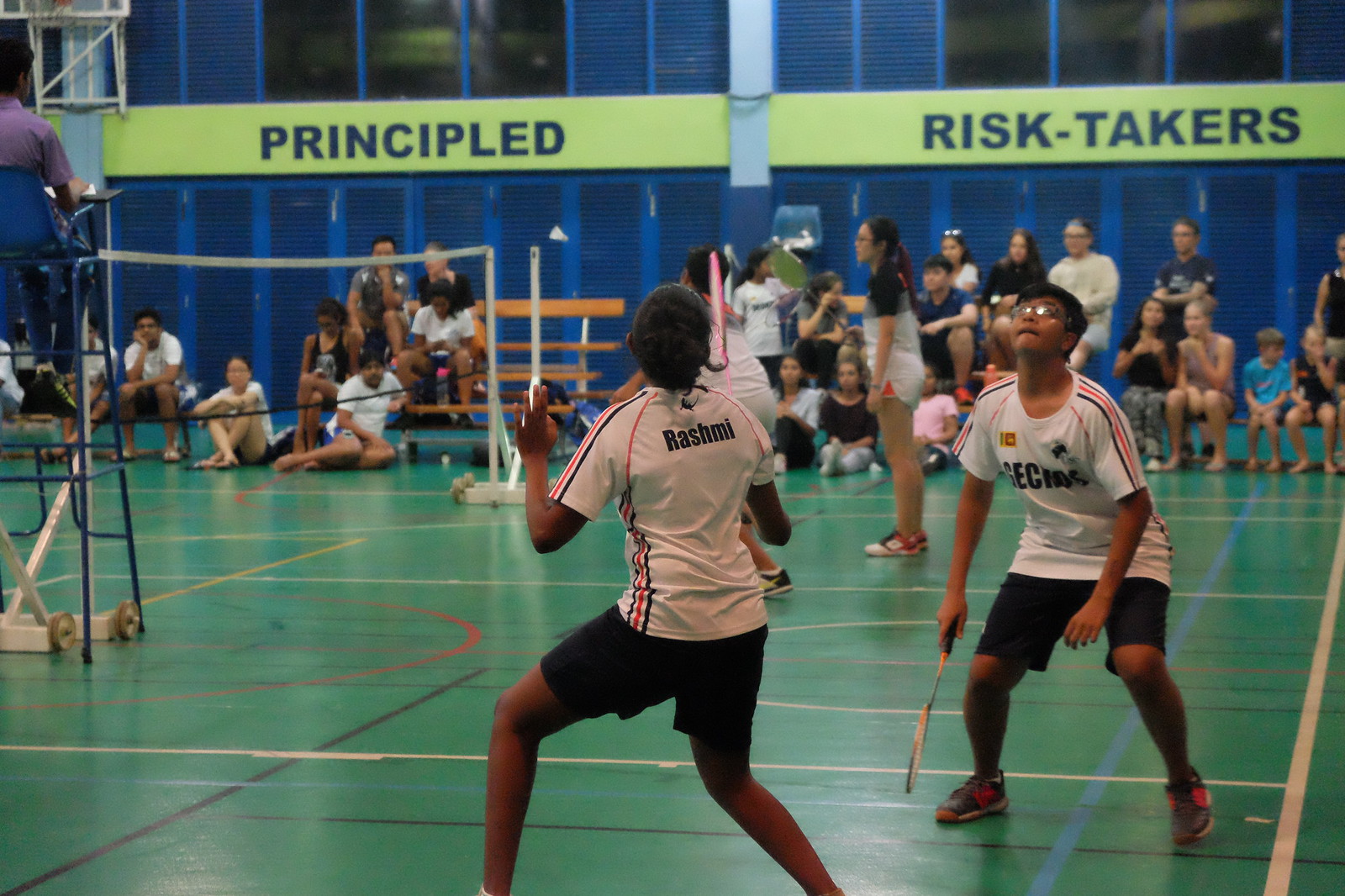The image captures an intense moment of a doubles badminton match set in an indoor gymnasium. The foreground is dominated by a green court with detailed boundary lines, suggesting it's a multipurpose sports floor. Two dark-skinned men, possibly in their teens or early twenties, are prominently featured, with both gazing upwards at an unseen shuttlecock. Each man holds a lightweight racket in their right hand. They are coordinated in white jerseys adorned with red and blue stripes on the shoulders and sides, paired with dark blue shorts. The player on the right, distinguished by his glasses, has his racket poised downward, seemingly waiting for his partner, whose back is to the picture, to make the next move.

To the left of the image stands a badminton net, demarcating the boundaries of the game. In the background, a variety of spectators, ranging from lighter to darker hues, are seated on benches, attentively watching the match. Above them hangs a substantial yellow banner with bold blue letters that read "Principled" and "Risk Takers." This banner sits just below a row of windows, indicating the gymnasium’s spacious, well-lit environment. The walls exhibit a pattern reminiscent of blue shutters or fencing, adding a unique aesthetic to the setting.